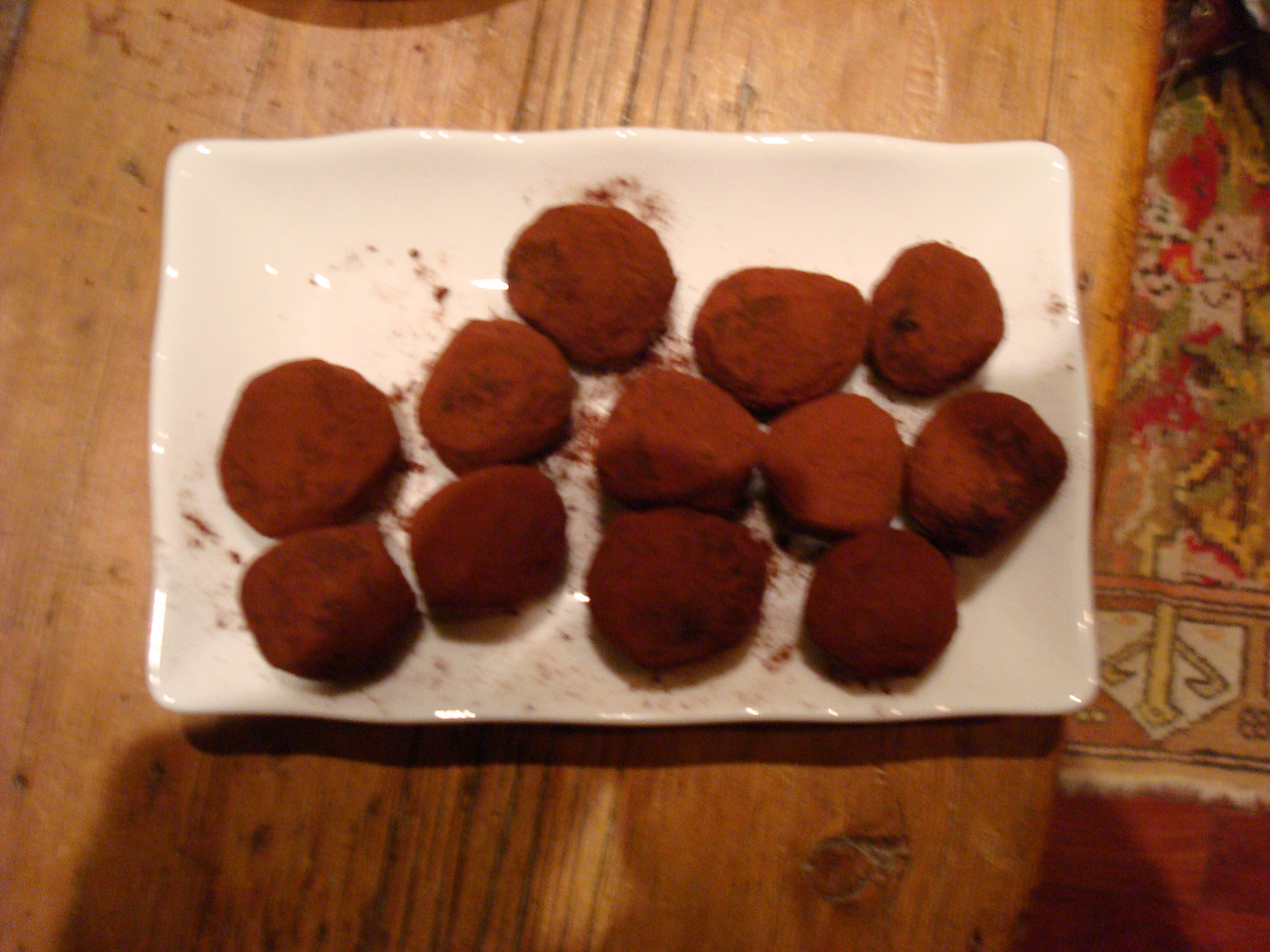This overhead photo captures a rustic scene featuring a small, white, scalloped platter placed on a pronounced wooden table with visible knots and intricate grain patterns. On the platter are twelve round-ish donuts, irregular in shape, generously coated in cinnamon and sugar. The wooden table appears to be of a lighter wood, possibly walnut, while on the right side of the image, part of an abstract-patterned rug with fine, short fringe is visible. The rug displays a harmonious mix of reds, greens, yellows, beige, and maybe brown, resting on a contrasting darker red wood floor. The photograph's lighting accentuates the texture of both the donuts and the table, casting subtle shadows, enhancing the overall cozy, rustic ambiance.